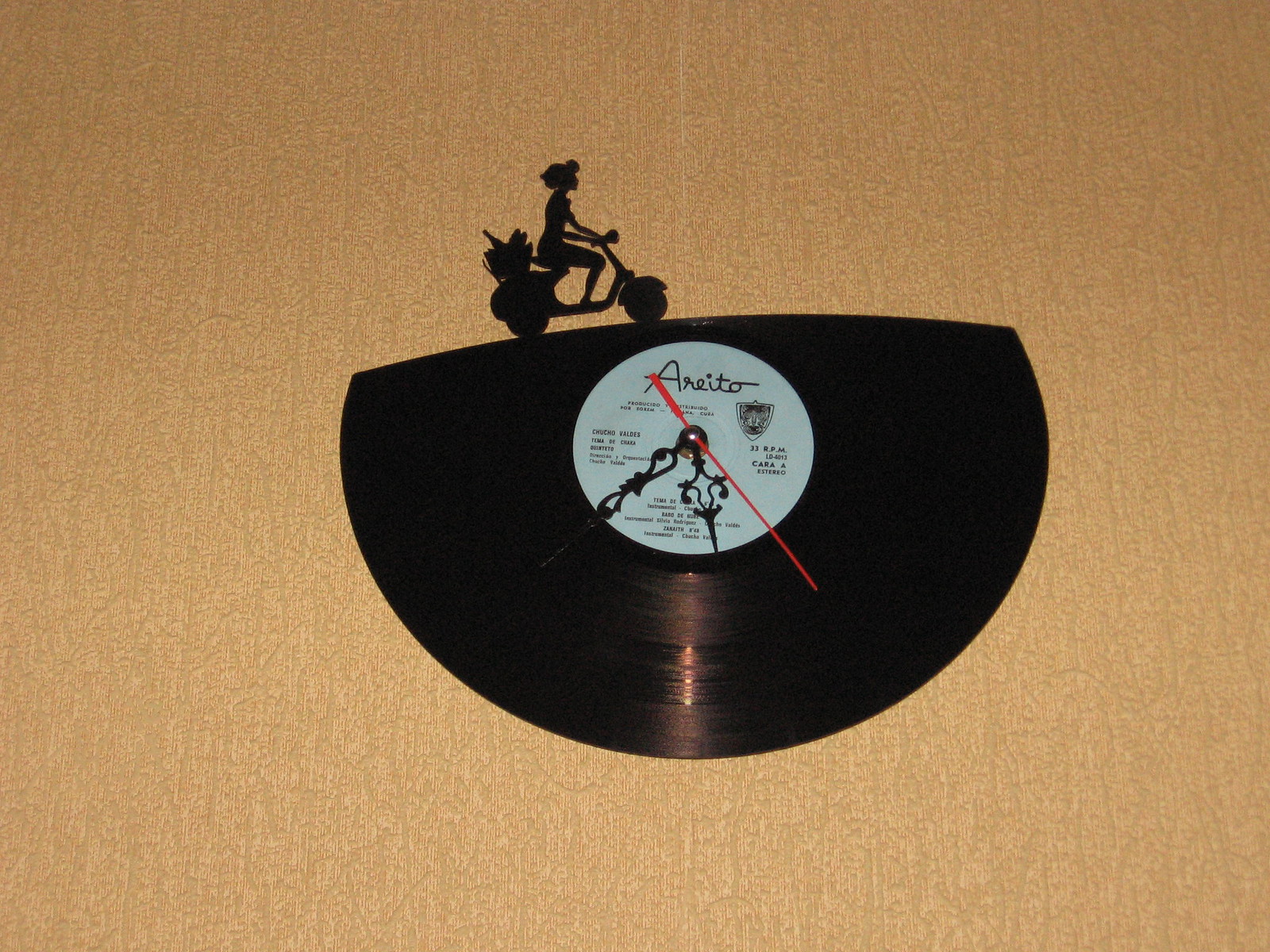This contemporary photograph showcases a distinctive clock crafted from a black vinyl record, which has been artistically transformed to embody a modernized Art Deco style. Central to the design is a light gray circular sticker featuring the brand name "ARIDIO" in cursive, along with other details too small to decipher. The clock face includes two black hands adorned with floral-like engravings and a red second hand, all set against a white inner circle of the record which is demarcated with 33 RPM and additional text.

Adding to its unique charm, the upper segment of the record is artfully cut out to reveal the silhouette of a woman with curled hair, dressed in a flowing attire, riding an electric scooter. The scooter is intricately depicted with visible tires, a front light, and a rear basket containing bread and possibly a bottle of wine. This black silhouette lacks intricate detail but stands out prominently against the light brown background upon which the entire composition rests. The artistic cutouts evoke the delicate precision of paper snowflakes, blending retro elements with a chic, contemporary twist.